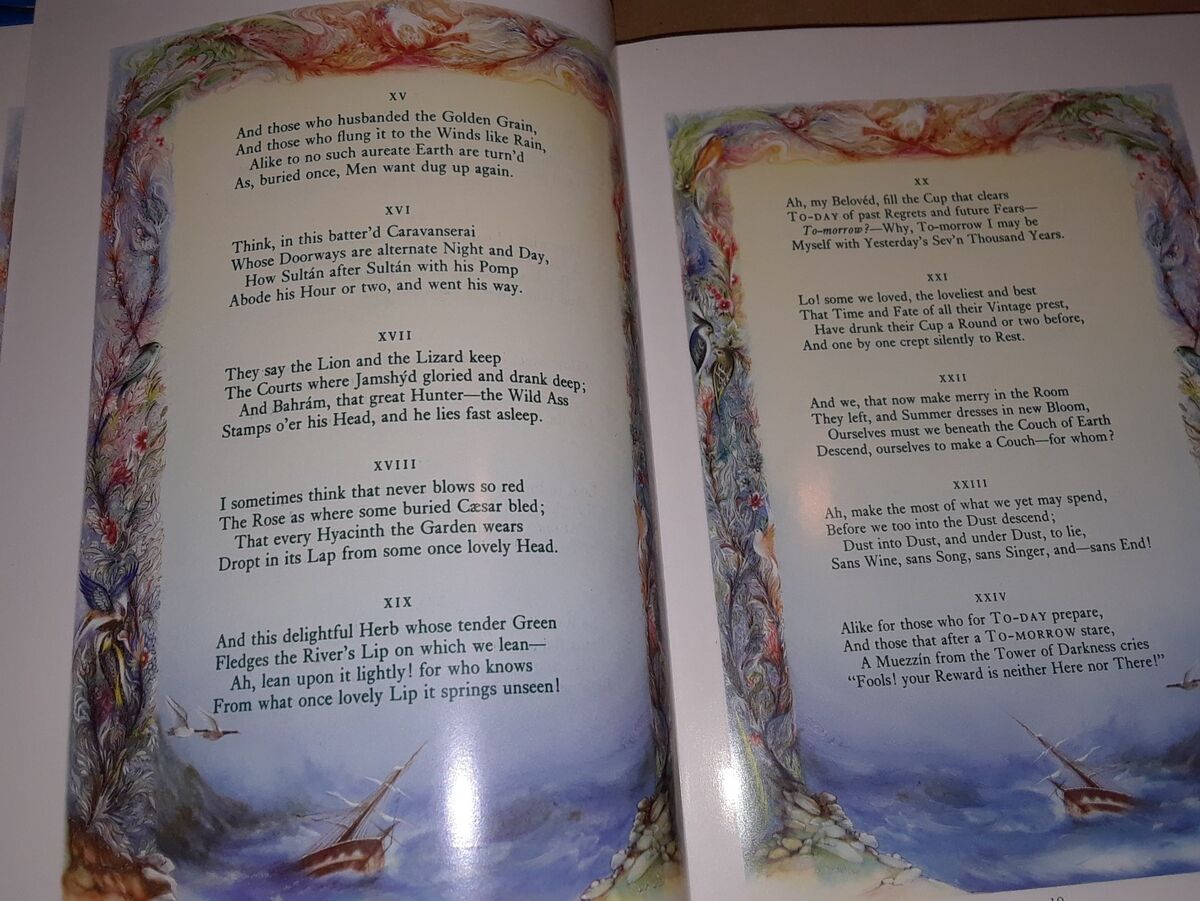The image captures an open book at its middle page, featuring glossy pages with a prominent white border adorned with intricate floral patterns and birds. The center of each page highlights a yellow background with black text; the left page begins with "XV" and contains verses that read, "and those who husbanded the golden grain and those who flung it to the winds like rain, alike to know such a re-earth are turnt, as buried once, men want dug up again." The succeeding passage, labeled "XVI," states, "Think, in this battered caravansary, whose doorways are alternate night and day, how Sultán after Sultán, with his pomp abode, his hour or two, and went his way." The border also incorporates water-themed elements like boats on the water and birds in flight, framing the text that stands out in what appears to be segments designated by Roman numerals.